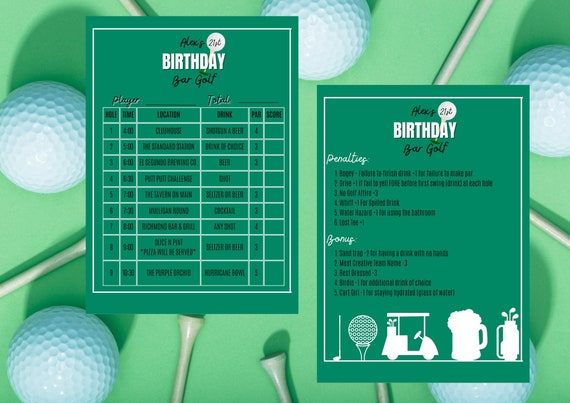This image features a detailed scorecard for "Alex's 21st Birthday Bar Golf." The background is a light green, scattered with five white golf balls and seven white golf tees. The scorecard is presented in two sections: the left one details the game setup, listing players, times, locations, drinks, pars, and scores. Various bars like the Purple Orchid and drinks like the Hurricane Bowl are mentioned. The right section includes additional information on penalties and bonuses, such as three extra points for being best dressed or for the most creative team name. Both sections have consistent headings with "Alex's 21st Birthday Bar Golf." The scorecards resemble birthday cards, adding a festive touch to this unique golfing celebration.